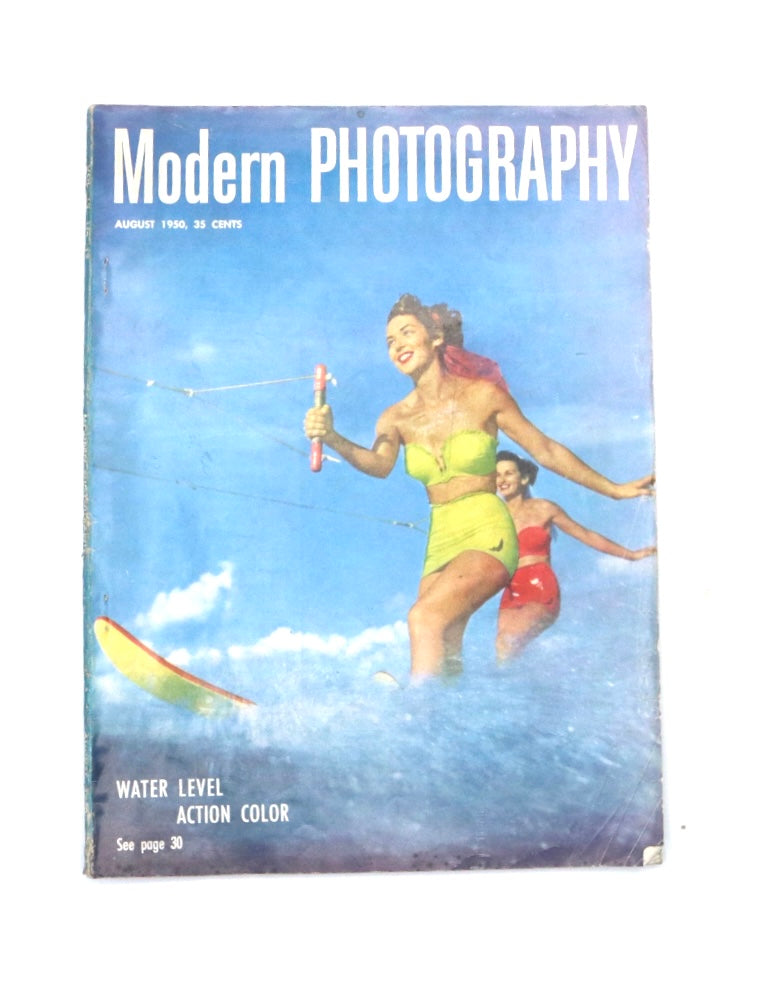The cover of the vintage magazine "Modern Photography," dated August 1930 and priced at 35 cents, features a vivid scene of two women water skiing against a backdrop of a light blue sky with subtle hints of gray clouds. In bold white text at the top, the title "Modern Photography" is prominently displayed. The foreground is dominated by a young woman with red hair, clad in a yellow two-piece bathing suit, smiling as she holds onto a water skiing tow rope with her left arm outstretched. Her outfit includes a short skirt and a bikini top, conveying the fashion of the era. Her legs, partially obscured by the splash of water, stand on a yellow and red-striped surfboard emerging from the frothy waves. 

Slightly behind her, another woman with short dark hair can be seen, dressed in a matching vintage red two-piece bathing suit. She too grips a water skiing tow rope with her right arm extended, balancing on a ski in the wake of their motion. The dynamic positioning of the women and the water splashing around them vividly captures the action and energy of the scene.

In the lower left corner of the cover, over the turbulent blue water, a white text reads "WATER LEVEL ACTION COLOR. See page 30." The magazine, although showing signs of wear and age, remains a striking example of mid-20th-century photography and style.